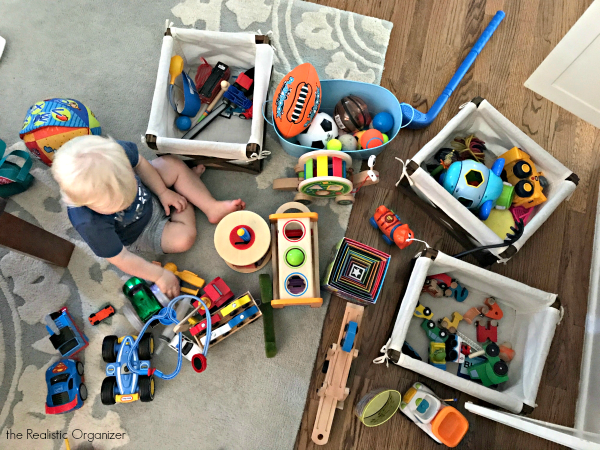In an overhead photograph of a young boy's playroom, a blonde-haired child, around four to five years old, is engrossed in playing with his toys. He's dressed in a blue shirt and gray shorts, sitting on a light blue and white rug placed over a wooden floor with a rich and varied grain. Surrounding him are various toy boxes, predominantly white with brown accents, filled with an assortment of cars and trucks in vibrant colors like yellow, blue, and red. A superhero logo is visible on one of the cars. 

Among the toys, there is a blue toy golf driver beside a basket filled with balls, including an orange football and a soft soccer ball. Other toys scattered around include race cars, construction equipment, a toy train, and even a spaceship. An open white door is visible on the right, hinting at the entrance to this cozy play area, which features a watermark in the bottom left corner reading "The Realistic Organizer." The boy appears deeply absorbed in selecting and playing with his treasured collection of cars and sports toys in his delightful, well-organized space.